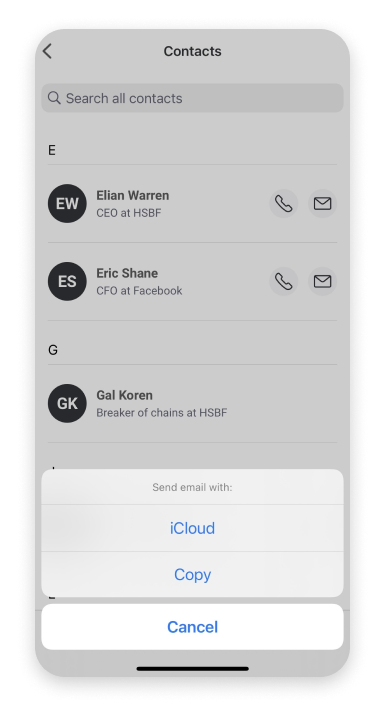The image appears to be a screenshot from a cell phone displaying the "Contacts" section. At the top of the screenshot, in a black banner, the word "Contacts" is prominently displayed. Just below this, there is a search bar labeled "search all contacts," allowing users to find specific contacts quickly. 

Underneath the search bar, the letter "E" is aligned to the left, signifying the beginning of contacts whose names start with E. Below this, there are two contact entries. The first entry shows Ellian Warren, identified as the CEO at HSAF. To the left of Ellian Warren's name is a black circle containing the initials "EW" in white. To the right of the contact name, there are two icons: a phone icon for making a call and an envelope icon for sending an email.

The second contact listed under the letter "E" is Eric Shane, titled as the CFO at Facebook. Adjacent to Eric Shane's name, there is a similar black circle with the initials "ES" in white, accompanied by the same phone and envelope icons on the right side.

As the contacts transition to the letter "G," the image displays a black circle with the initials "GK" next to the name Gal Coren, who is labeled as the "Breaker of Chains" at HSBF, followed by the same set of phone and envelope icons.

Beneath the contacts, a prominent white pop-up rectangle emerges, contrasting with the gray background. This pop-up contains an instruction to "send email with" followed by two blue options: "iCloud" and "copy." Below these options, there is a separated bar labeled "cancel," allowing the user to dismiss the pop-up.

The screenshot meticulously captures the layout and various elements of the phone's contacts interface, highlighting the names, titles, initials, and available communication options.